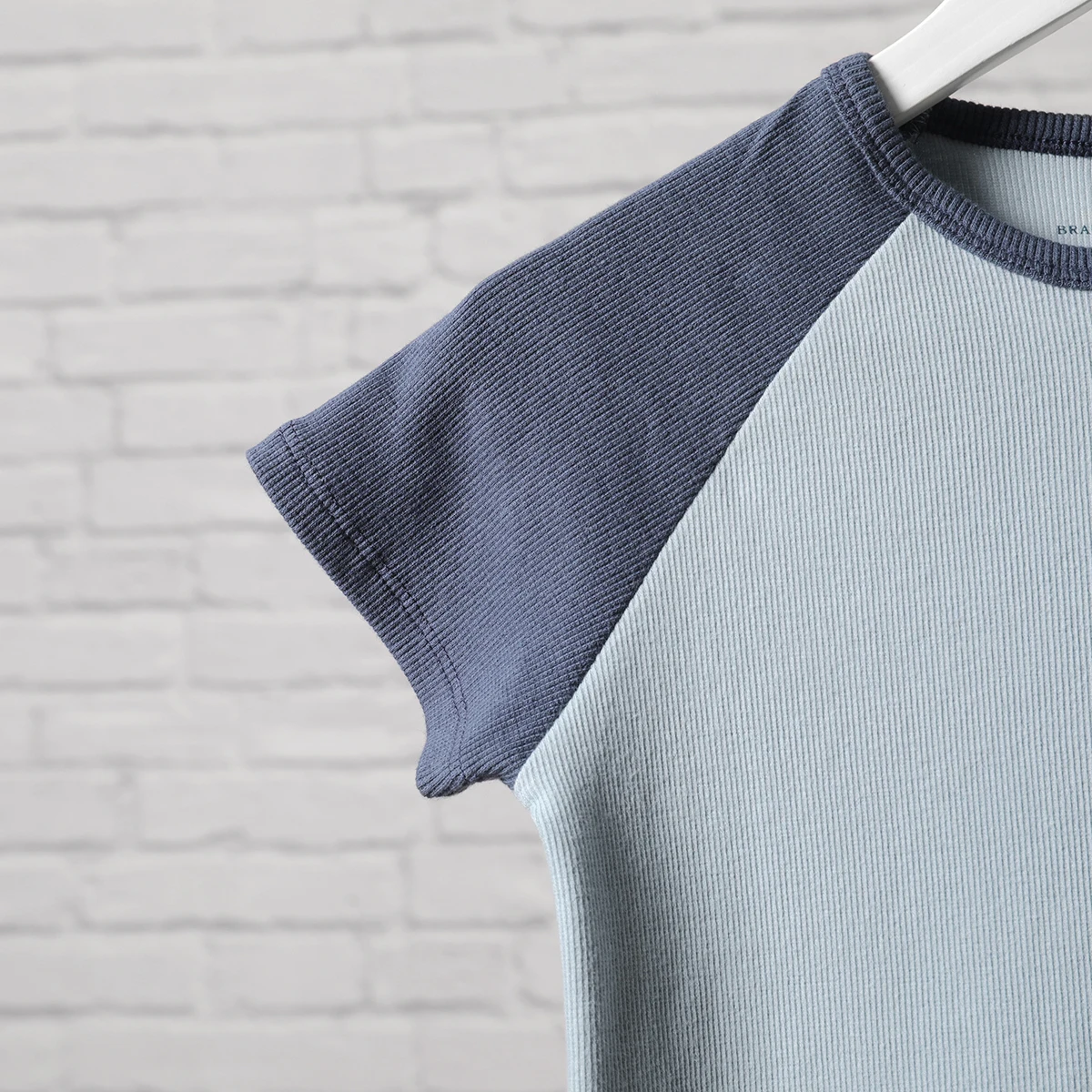The image depicts a portion of a short-sleeve t-shirt hanging on a white hanger against a slightly blurred white brick wall. The shirt features a two-toned design with a dark gray collar and a dark gray sleeve, while the rest of the shirt appears to be a lighter gray or possibly blue. The shirt has a vertical texture running down the fabric, implying it is sewn with visible thread lines on the shoulder. In the upper right corner of the image, part of the hanger is visible. The shirt's tag is partially visible, with the letters "B-R-A" printed inside, though the rest of the tag is cut off due to the framing of the picture. Additionally, a shadow is cast on the left side of the shirt (our right). The entire picture is square and has no border, and only the upper half of the shirt is shown.